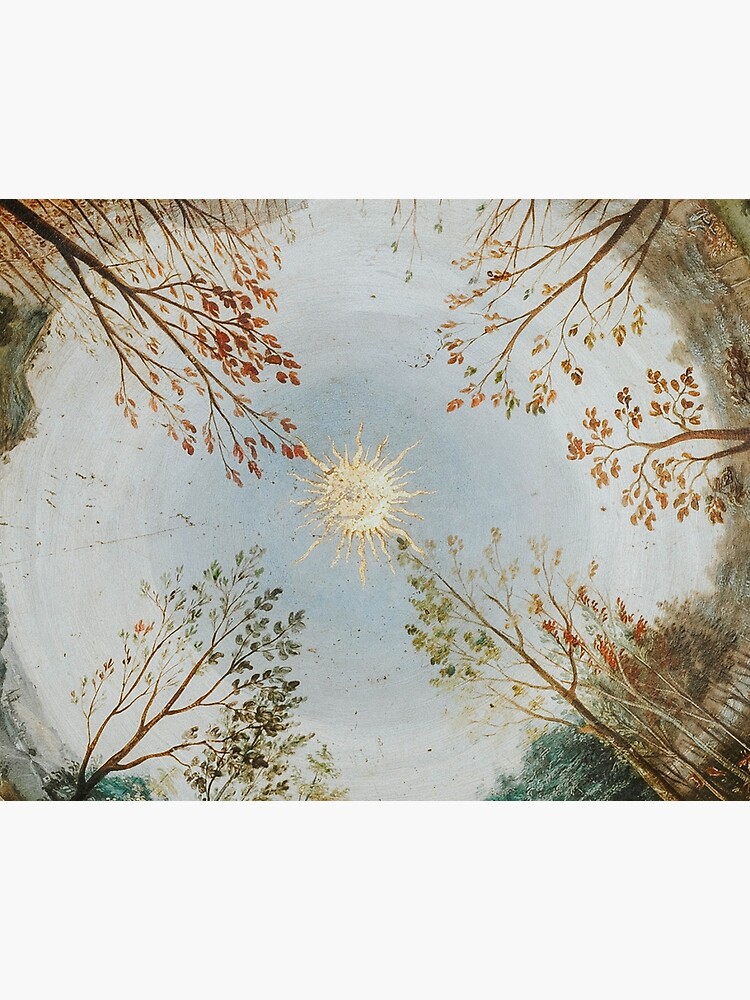This detailed painting captures a stunning 360-degree view from the ground, looking up towards a bright yellow sun emitting scattered rays that dominate the center of the circular image. The sky transitions from a gradient blue with hints of gray. Surrounding the sun are various trees, their tall, narrow, and wispy branches reaching upwards. The foliage presents a vibrant palette indicative of fall: lush greens, vivid oranges, deep reds, and rustic browns. Each tree appears unique, adding diversity to the scene. Beneath this colorful canopy, the ground foliage also hints at autumn with hints of browning grass, enhancing the seasonal feel. Beyond the immediate trees, a dense forest of green and brown trees extends into the horizon, encapsulating the viewer in this serene woodland setting.